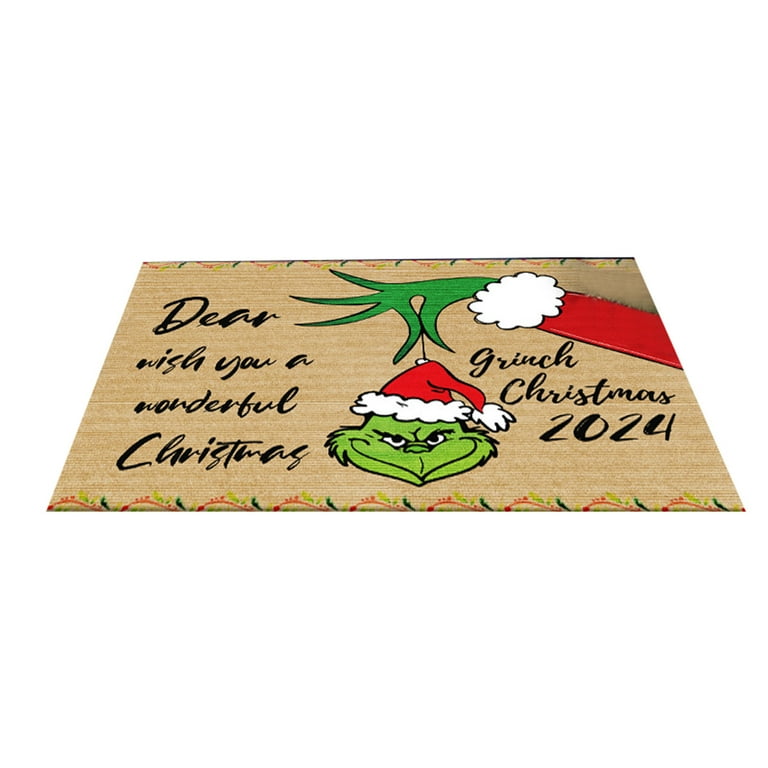The image depicts a beige, rectangular doormat with a rattan-style texture. The design features a festive, Grinch-themed motif. On the left side, in black lettering, it reads, "Dear, wish you a wonderful Christmas." The center showcases the Grinch's pinched thumb and index finger, holding an ornament that resembles his green, smirking face, complete with a classic red and white Santa Claus hat. His hand extends from a red-sleeved arm with a white cuff, and the thin string suspending the ornament is visible between his fingers. On the right side, cursive lettering reads, "Grinch Christmas 2021." The mat is bordered by green and red squiggly lines, and the background of the image is white, suggesting it may have been digitally edited. There is a slight blur in the top right corner of the mat.